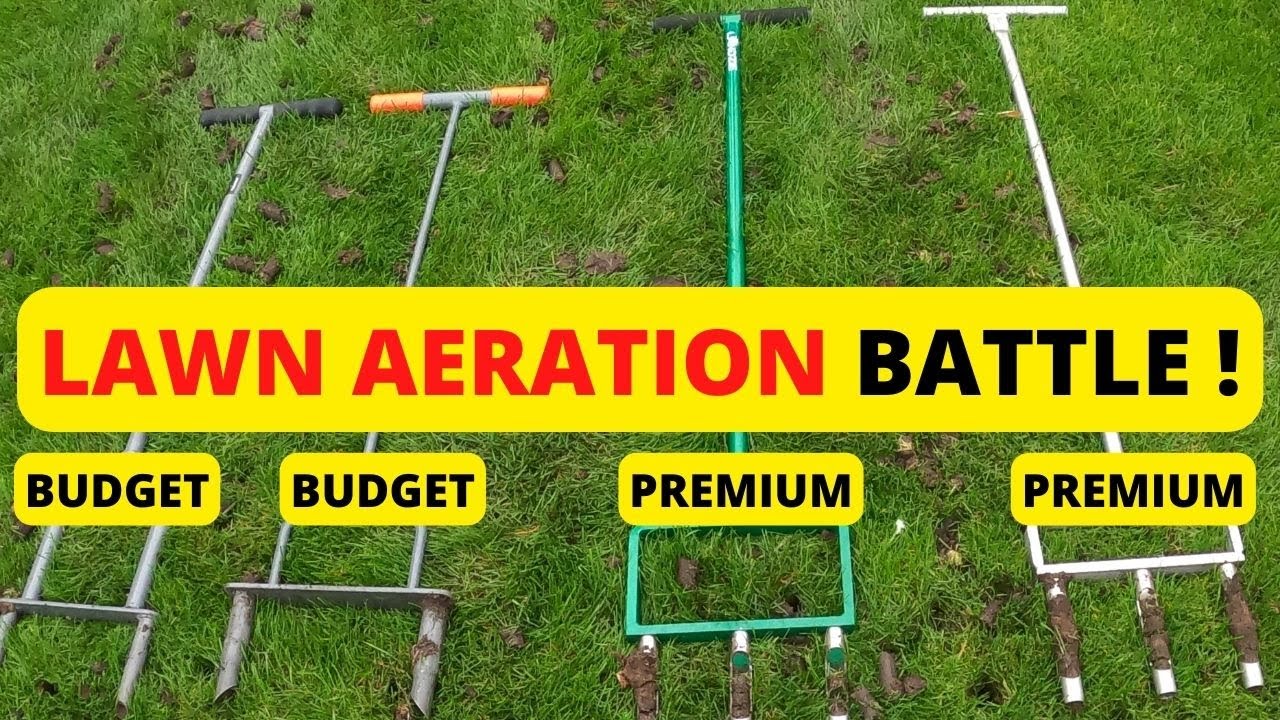The image depicts a vibrant green lawn with some brown patches, possibly fertilizer, and prominently features an advertisement with the text "Lawn Aeration Battle" against a yellow background. The words "Lawn Aeration" are in red, while "Battle" is in black. Below this text, four garden tools, believed to be for lawn aeration, are laid out horizontally on the lawn. Each tool has a handle, a long shaft, and a unique design at the end. The two tools on the left are labeled "Budget" and differ as follows: one has a black handle and two straight metal tubes, while the other has an orange handle with slanted tubes. On the right side, the "Premium" labeled tools feature three blades or tubes and are colored green and white, respectively. The purpose of these tools is likely to poke holes in the lawn to aerate the soil.